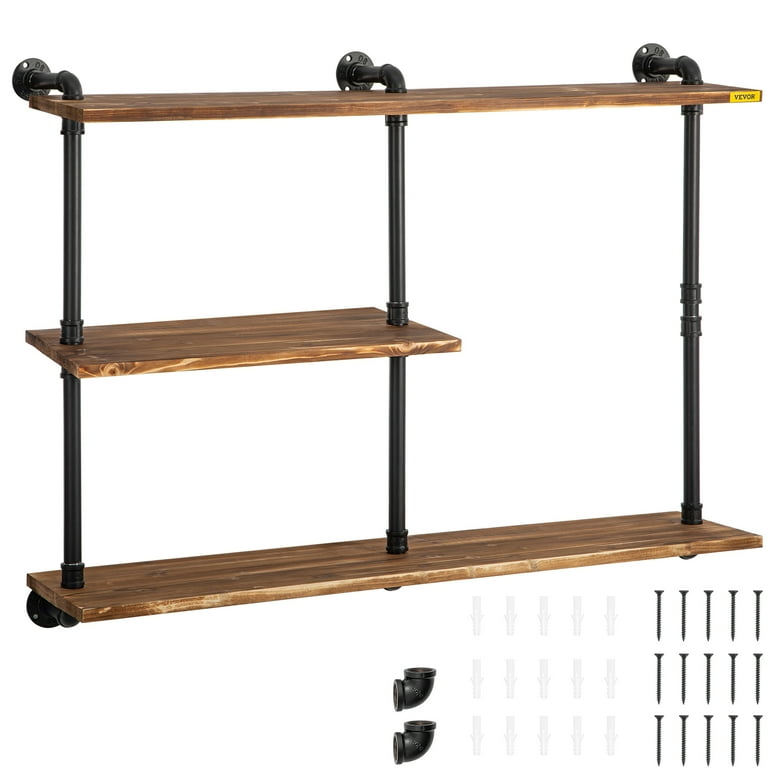This image features a rustic-style wall shelf made up of three wood shelves, supported by black pipe fittings designed to look like iron. The top and bottom shelves are long and extend across the entire frame, while the middle shelf is half the length of the other two. Each shelf is connected by three black metal pipes running vertically through the ends, which are flattened into circles with holes for wall mounting. The image includes additional components such as pipe ends, screws, and wall anchors necessary for installation. The background is white, enhancing the contrast of the brown wooden shelves and black piping. In the upper right corner, there is a label that reads "VEVOR."